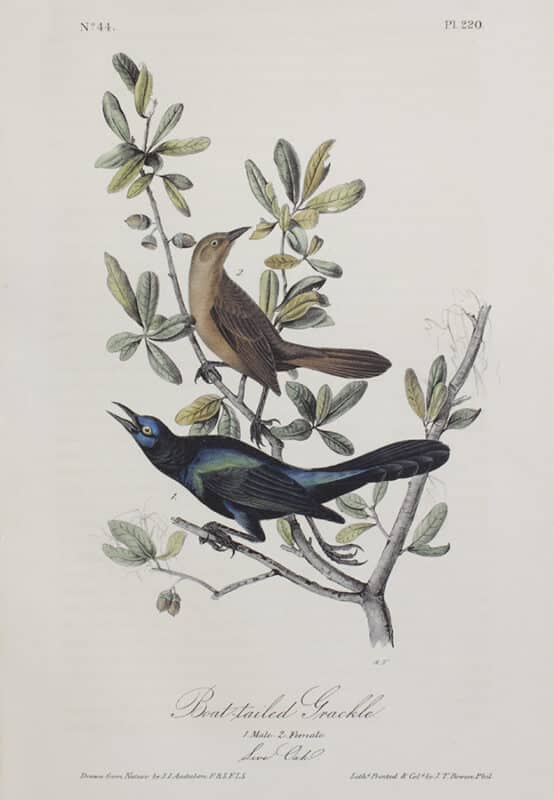The image is an artist's rendition of two grackles perching on branches. The main subjects are a pair of birds detailed with delicate, old-illustration-like precision. The background has an off-white coloration, reminiscent of an aged etching or print. There are thin twigs and some green leaves among the branches. At the top, the numbers "44" and "P220" are inscribed on the upper left and right corners respectively.

The bird on the lower half of the image, identified as male by a number "1" beside it, is mostly black with iridescent blue and green accents on its wings and face. It appears to be cawing while looking upwards. The bird on the upper branch, facing left but looking right, is smaller and predominantly brown with a tan body and a darker brown back, suggesting it to be female.

Beneath the artistic depiction, there's slightly blurry text in a centered, scripted font that reads, "boat-tailed grackles," though it's hard to discern clearly. The overall white page only features artistic elements and inscriptions, giving it a minimalistic yet detailed appeal.